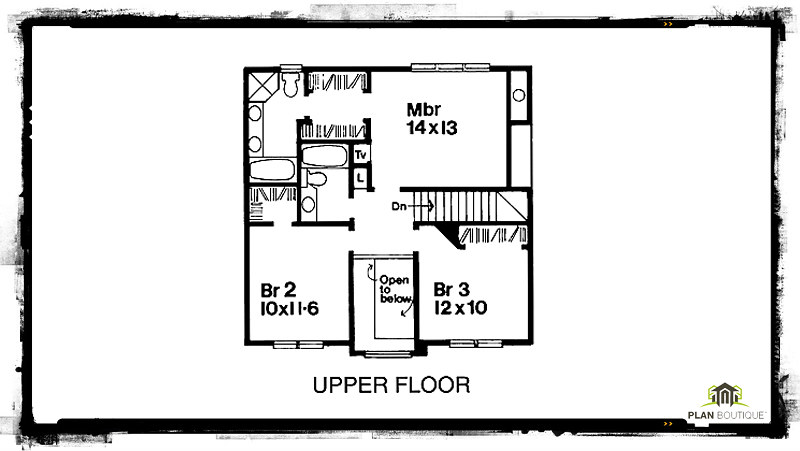This detailed blueprint image illustrates the floor plan of a boutique-style house. The image is framed within a streaky, black-inked rectangle. At the bottom right, there is a small emblem reading "Plan Boutique" in black text accompanied by a black outlined icon of a house surrounded by a greenish hue.

Central to the blueprint is the main floor plan, intricately detailed in black ink. The floor plan itself is enclosed within a square outline. The layout specifies various rooms and features:

- **Bottom Left**: An area labeled "BR2" (Bedroom 2) measuring 10x11-6, marked as an empty space.
- **Middle**: A vertical rectangle indicating an open area labeled "Open to Below."
- **Beside the Open Space**: Another empty spot designated as "BR3" (Bedroom 3), measuring 12x10.
- **Top and Middle**: Just above and centrally located is a staircase marked "Staircase Down."

**Top Section**:
- Positioned in the upper middle section is a space labeled "MBR" (Master Bedroom), measuring 14x13, and marked as an empty space.

**Left Section**:
- Adjacent to the MBR to the left are several objects of varying shapes, including rectangles and ovals, with labels such as a square reading "TV" and another marked "L" underneath it. 
- **Top Left**: A small compartment identifies a toilet area.
- **Middle Left**: There is another square seen, suggesting another toilet area below it, alongside a circle that likely represents a sink.

This intricate layout presents a clear and functional design of the floor space, offering a comprehensive understanding of the room distributions and their respective dimensions.